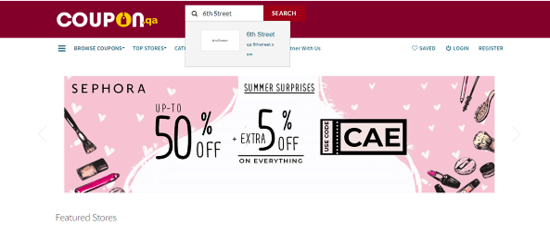The top left corner of the image features the "coupon.qa" logo, with the second "O" creatively designed as a yellow price tag icon. This logo is placed within a red banner. Immediately to the right of the logo is a search bar labeled "6th Street," accompanied by a red search button. Beneath the search bar, there's a blue text drop-down menu that also reads "6th Street".

Below these elements, on a white background, are several blue headlines titled "Browse Coupons," "Top Stories," and more, although some of these headings are partially obscured by the drop-down menu. On the right-hand side of the white section, blue text indicates options for "Saved," "Login," and "Register."

The bottom portion of the image showcases an advertisement for Sephora. At the top left of this ad, the Sephora logo appears in black text. The ad promotes "Summer Surprises" with discounts of "up to 50% off" and an additional "5% off on everything," provided shoppers use the code "CAE". 

This Sephora ad is set against a pink background adorned with white heart patterns. To the left side of the ad, there are various makeup items, including brushes, lipstick, and a hairbrush. Below the Sephora promotion, there is a "Featured Stores" section.